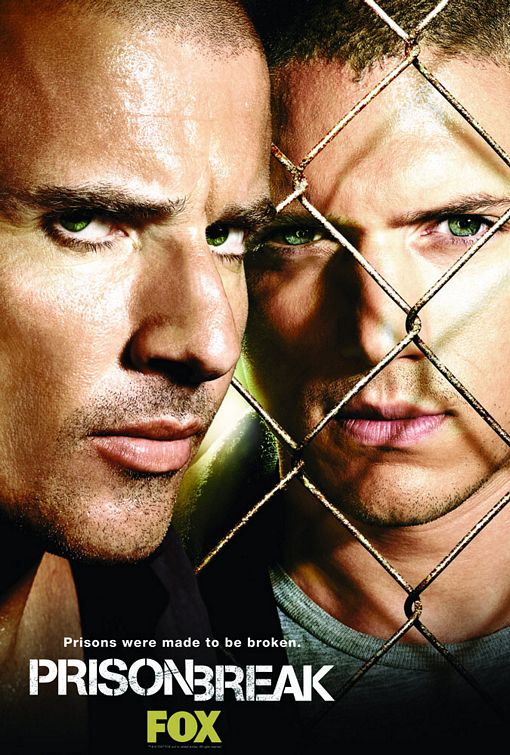The poster for the TV show "Prison Break" on Fox features a close-up of two men's faces, emphasizing their intense and scowling green eyes. Both men have short, dark brown hair and stubbled facial hair, with one man positioned behind a chain-link fence and the other in front of it, symbolizing the theme of imprisonment and escape. The man on the right side appears slightly more tanned, adding to the intense and rugged look. Their furrowed brows and piercing stares further add to the dramatic feel of the image. In the bottom left, white text reads, "Prisons were made to be broken," followed by the show's title, "Prison Break," in a distinctive blocky font, with "Fox" written underneath in olive green text. Their close-cropped hair and minimal visible parts of their necks and chests hint at a deliberate stylistic choice reflective of their characters' struggles and the gritty atmosphere of the show.